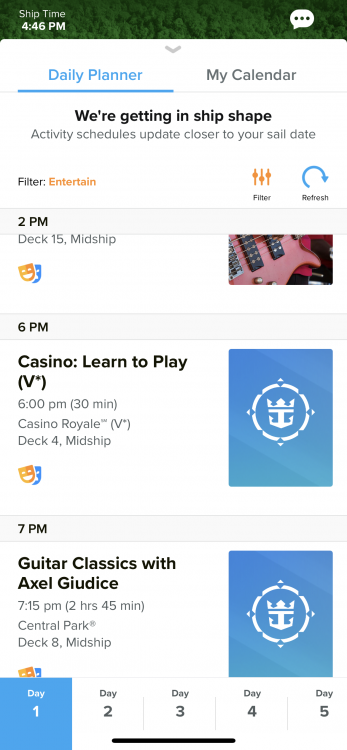The image depicts a smartphone screenshot of a daily planner app titled "My Calendar," which appears to be catering to cruise ship guests. The interface is clean and modern, with clear text and bold headers. A notification at the top reads, "We're getting in ship shape. Activity schedules update closer to your sail date," indicating that the details might be subject to change. 

Among the activities listed:

- **2:00 PM:** An unidentified event taking place on Deck 15, Midship.
- **6:00 PM:** A "Casino Learn to Play" session starts, lasting for 30 minutes at the Casino Royale, located on Deck 4, Midship.
- **7:15 PM:** "Guitar Classics with Axl Geodes," a musical performance that spans 2 hours and 45 minutes in Central Park on Deck 8, Midship.

This schedule is for day one of a five-day itinerary. The current time shown is 4:46 PM ship time, and the app's interface includes three dots in the top right corner, likely for additional options or comments. This detailed layout helps passengers plan their day with ease and enjoy their cruise experience.